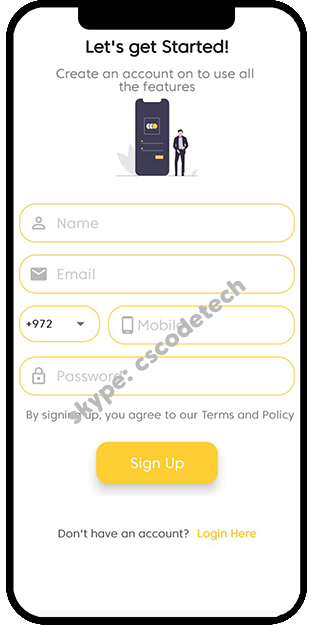The image features a black cell phone set against a pristine white background. Displayed prominently on the phone's screen is a website interface. At the top of the screen, in bold black text, it reads, "Let's get started." Beneath this, a subheading instructs users to "Create an account to use all the features."

To the right of the phone, a male figure is standing, adding a human element to the scene. Below the instructional text on the phone's screen, there is a yellow, lined form with fields for name, email, and a dropdown button pre-filled with "+972." Following these form fields is a prominent yellow action button labeled "Sign Up."

At the bottom of the display, in small dark gray text, a message reads, "Don't have an account?" To its right, in yellow text, is an interactive link, "login here."

Adding a tech-savvy aesthetic, the words "Skype CS Code Tech" are diagonally superimposed across the image, running from the lower-left corner to the upper-right corner in subtle gray text.